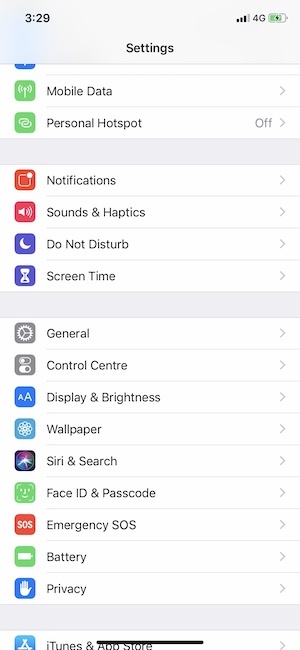The image is a vertically-oriented rectangular screenshot of an iPhone's settings menu. At the top, there's a white status bar displaying the time as 3:29, with "Settings" indicated prominently. On the left side of the status bar, there is a signal strength indicator showing three out of four bars, and a '4G' symbol next to it. To the right, a battery icon indicates a 75% charge. 

Below the status bar, the main settings menu begins. The first section includes options for "Mobile Data" and "Personal Hotspot" (not activated), separated by a gray divider spanning the width of the screen. The next section lists settings for "Notifications," "Sounds & Haptics," "Do Not Disturb," and "Screen Time," followed by another gray divider. 

Continuing down, the settings menu shows options for "General," "Control Center," "Display & Brightness," "Wallpaper," "Siri & Search," "Face ID & Passcode," "Emergency SOS," "Battery," and "Privacy." Each option has a rightward-pointing arrow, indicating further customizable settings within each section. The visible part of the menu ends with "iTunes & App Store," only partially visible, suggesting more options are available further down.